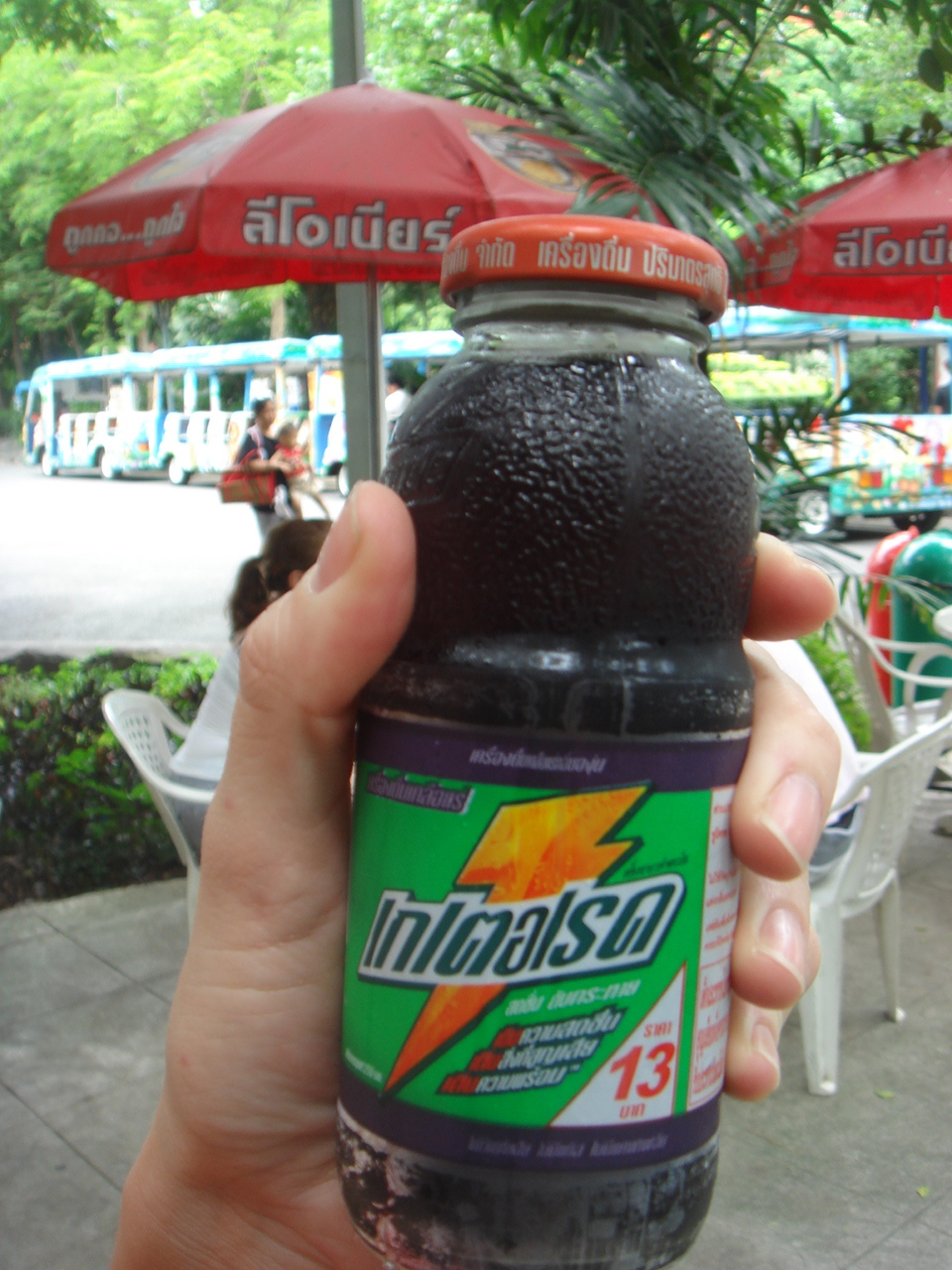The image depicts a glass bottle of a dark purple beverage, resembling Gatorade with its distinct green label and orange-yellow lightning bolt logo, though the writing is in an unfamiliar foreign language. The bottle, held by a light-brown-skinned male's left hand with well-manicured fingernails, features a round red lid with white writing. The background reveals a tropical outdoor setting with red umbrellas shading white plastic tables and chairs, some with foreign inscriptions. Directly behind the hand, a woman with a ponytail is seated. Further back, trees and a tram, possibly from an amusement park, can be seen against the gray concrete ground.